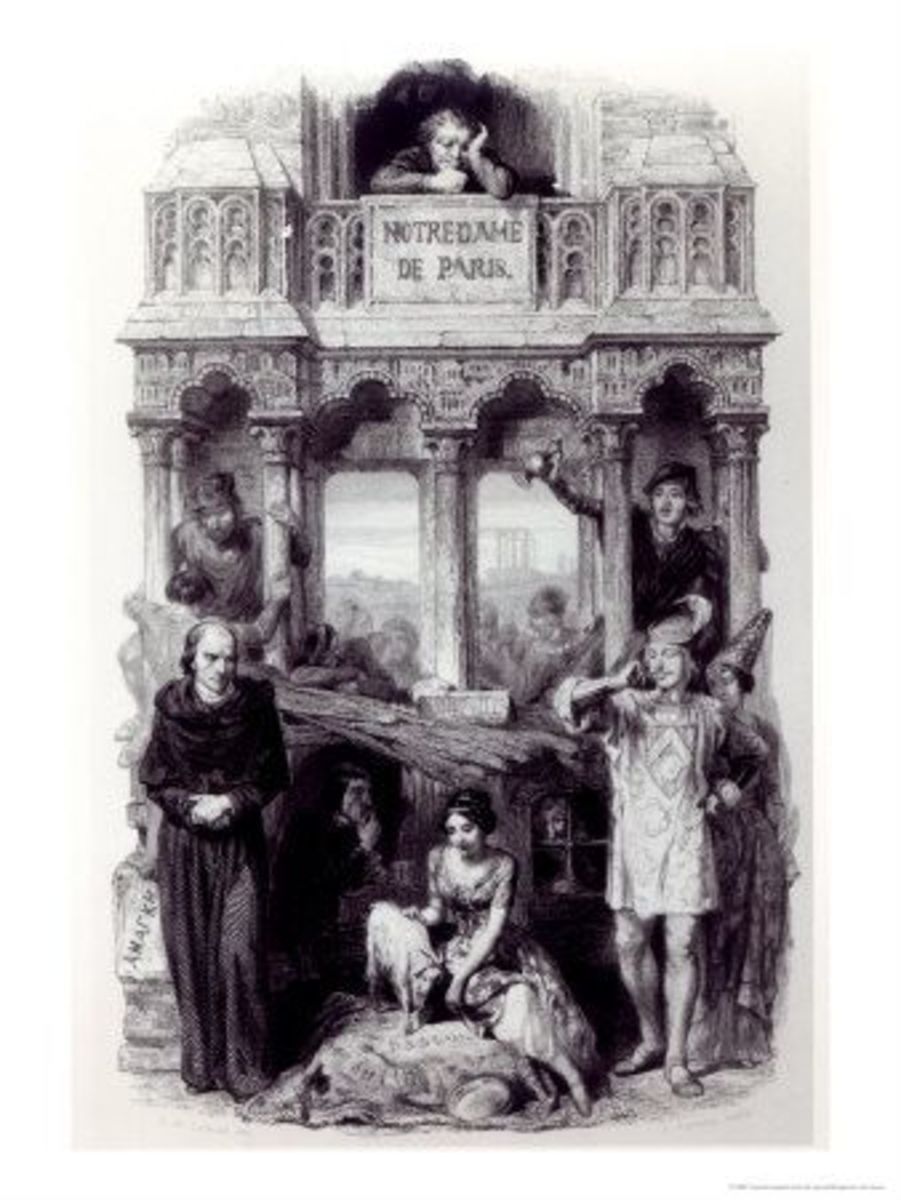This intricate black and white sketch portrays a scene set against the iconic backdrop of Notre Dame de Paris. The artwork, seemingly sketched with pencil or charcoals, captures an old-world ambiance. The composition, taller than it is wide, features a prominent architectural structure with two small archways and a sign above that reads "Notre Dame de Paris." Just above the sign, a melancholic figure leans over a balcony, head resting in hands, evoking the image of Quasimodo from Victor Hugo's novel.

Below this somber character, the scene is bustling with various individuals. On the right, a foreboding man clad in a black friar’s cassock stands, his presence contrasting sharply with the more whimsical elements in the sketch. Central to the composition is a woman garbed in a flapper-style dress, seated on what appears to be a fabric-draped rock. To her left, a small goat seems to rest, adding a pastoral touch to the scene. Flanking this central scene, two figures to her left are dressed in attire reminiscent of a court jester and a princess. The overall atmosphere is one of a historical tableau, teeming with diverse characters and rich in period detail.